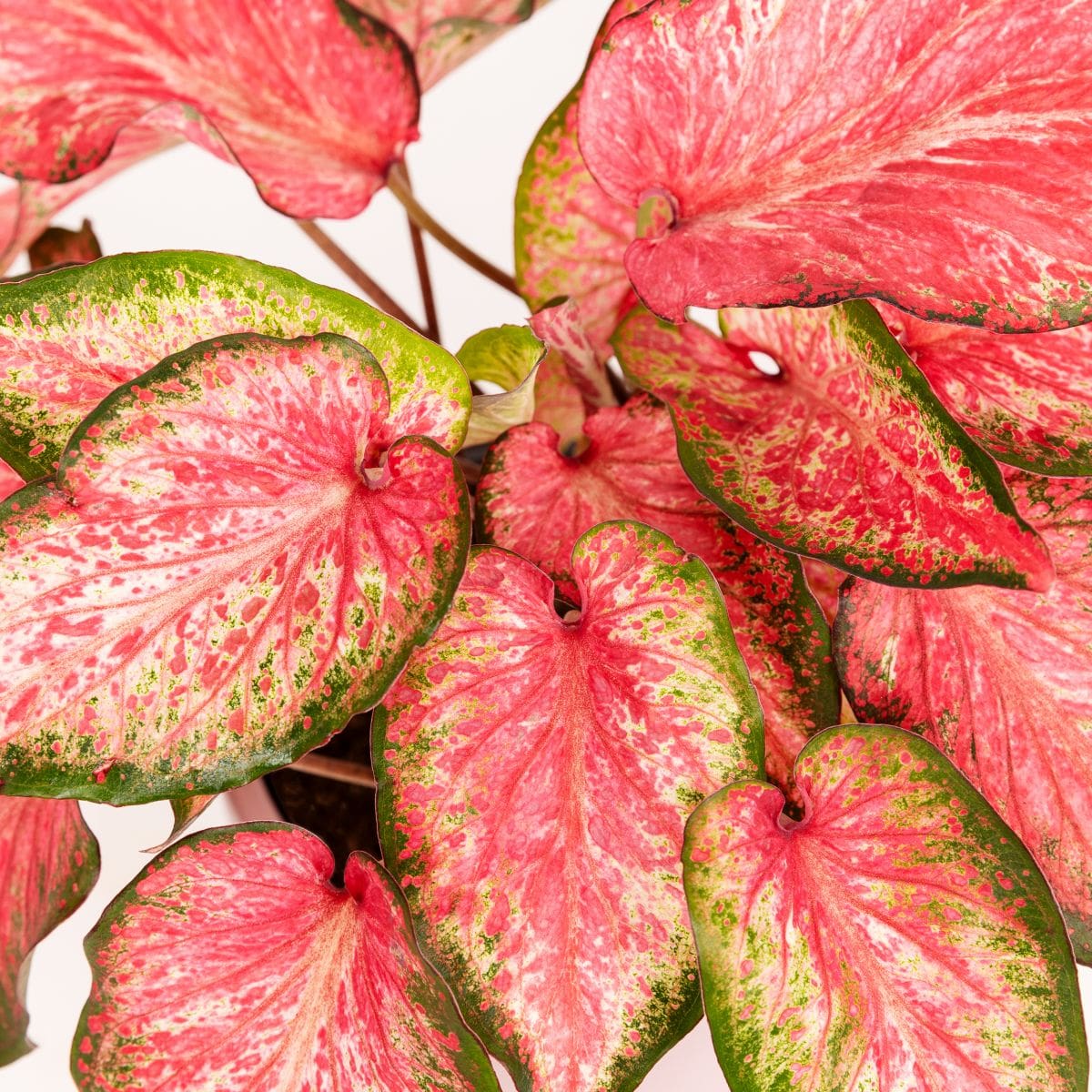This image captures a detailed close-up of a collection of plant leaves, possibly poinsettias, arranged against a pristine, solid white background with no visible flowers or fruits. The leaves are the central focus, displaying a variety of colors and patterns. Predominantly, they feature light pink to dark pink hues, accented with green borders, and some of them transition to white towards their tips, creating a striking visual contrast. The leaves are tall rather than wide, with light brown stems subtly positioned among them. The image reveals roughly 15 leaves, some overlapping and others spaced out. Leaves in the bottom right and middle sections are more densely packed, whereas the top left shows more spacing. Additionally, the lower left of the frame hints at the white side of a pot filled with dirt, indicating that the photograph might have been taken from a top-down perspective. Overall, this meticulous arrangement and color variation in the leaves, captured on a white backdrop, highlights their intricate patterns and natural beauty.